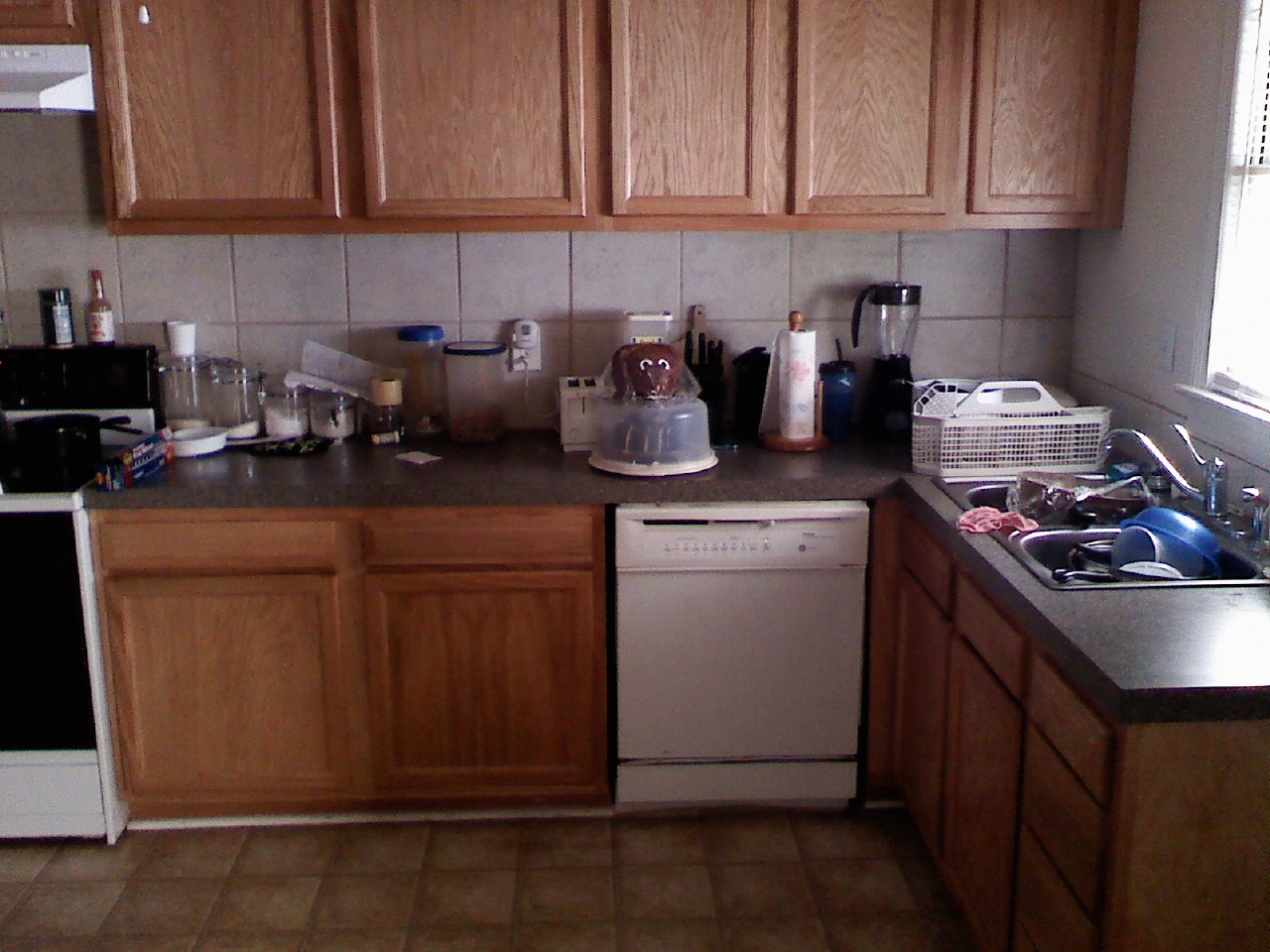A detailed image of a cozy kitchen interior showcases several oak or maple wood cabinets, including five upper and five lower ones, though more may be out of frame. The countertops, possibly black granite, are cluttered with kitchen essentials. The sink brims with dishes, including a prominent blue dish among several others, while a dish rack, blender, paper towel holder with a roll of paper towels, and jars of spices and baking ingredients occupy the surrounding space. Additional items like sauce bottles, a toaster, and an aluminum foil roll are visible, enhancing the kitchen's lived-in feel. To the left, a white and black oven is seen, with pots placed on the stove, completing the bustling kitchen scene.